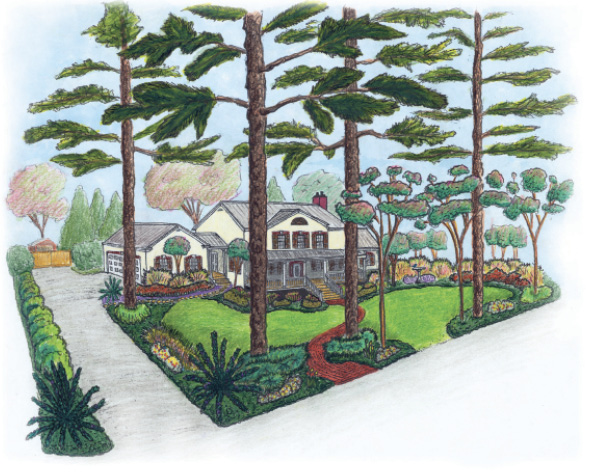This highly detailed illustration captures the essence of a charming, older-style light yellow house with intricate landscaping. The house, adorned with dark brown shutters and a gray roof, features a brown chimney peeking from the back. A prominent feature is its long, inviting porch which spans the width of the house and is accessed by approximately 10 to 15 stairs, depending on the interpretation, winding up from the lush yard.

To the left of the house, a garage with matching light yellow walls and dark brown shutters is connected to the main structure via a small walkway. The long, red-tinged driveway stretches from the street up to the garage. On either side of the driveway, a row of round-shaped shrubs and distinctive green plants resembling spider legs weave a natural border. The detailed landscaping includes more than five different species of flora, creating a vibrant garden-like ambiance. The left side features a storage house behind a yellow fence, painted red and complemented by the tall trees in the background.

Tall, thin trees line the front closer to the street, with a total of four tall trees and three smaller ones dotting the front yard. Additional tree life enhances the greenery in the background. Beautifully arranged flowers and smaller shrubs surround the base of a prominent tree to the right of the driveway. Paths zigzag in an S-shape leading to the porch, adding a dynamic flow to the overall landscape design. The intricate detailing of the home’s structure, combined with the lavish and colorful landscaping, all contribute to the picturesque beauty of this house, making it an inviting and warm dwelling.